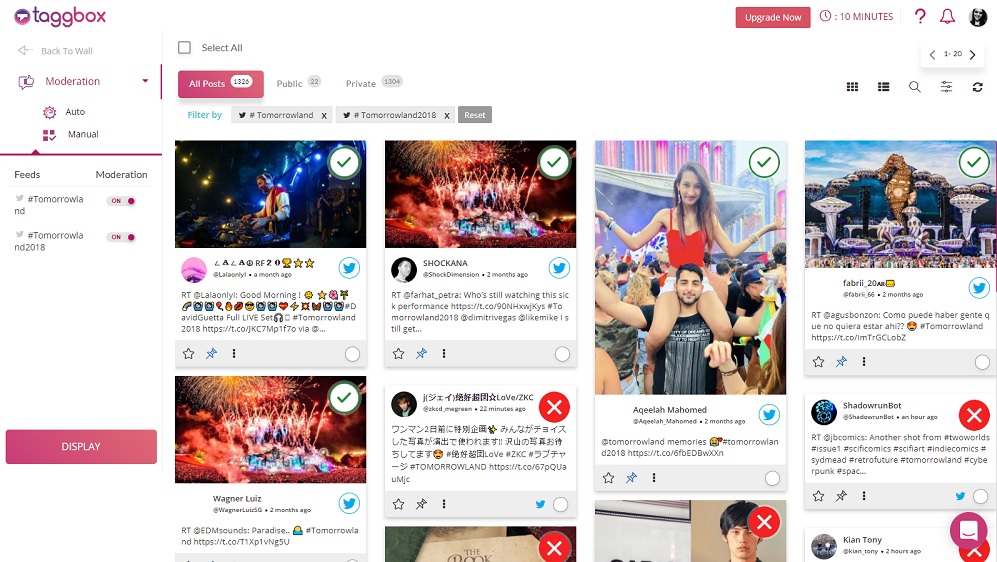On the Tagbox website, the background is predominantly white with accents of mauve and light pink hues. At the center of the webpage, an array of images is displayed, varying in size and vividly capturing celebratory scenes. Notably, some photos feature fireworks in full splendor. Another striking image shows a young man and woman at a concert, with the woman seated on the man's shoulders, both appearing to be in their youthful prime and of Caucasian descent. On the left-hand side of the page, a navigation bar is present. At the top of this bar, there is an option labeled "Back to Wall" accompanied by an arrow. Further down, there is a moderation section offering options for either automatic or manual moderation. Additionally, within the feeds section under moderation, there is an ombre box transitioning from mauve to light pink with the word "Display" prominently written in white at the bottom.